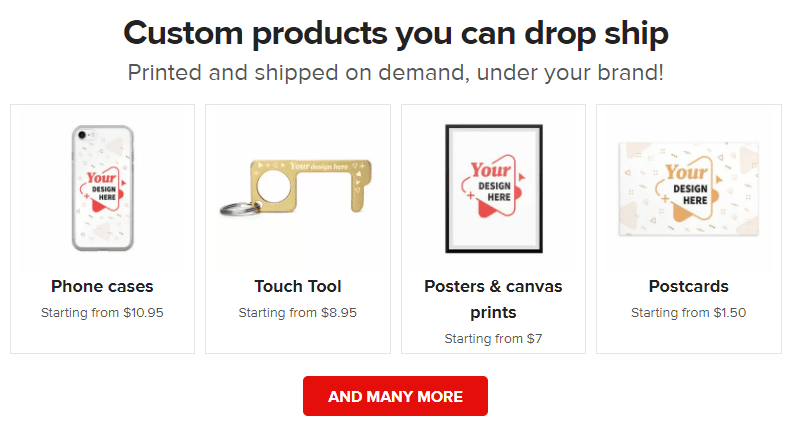The image displays a promotional banner with prominent bold text at the top reading "Custom Products You Can Drop Ship." Below this, in a smaller, lighter gray font, it states, "Printed and shipped on demand under your brand." The main section features four distinct boxes outlined in a subtle gray border. Each box showcases a different product with the text "Your Design Here," emphasizing customization options. The items include:

1. A phone case labeled "Phone Cases" with a starting price of $10.95. It features a red design template.
2. A touch tool described as "Touch Tool" with a starting price of $8.95, pictured as a golden keychain-like item.
3. A frame labeled "Posters and Canvas Prints," with prices starting at $7.00, showing as a customizable picture frame.
4. A postcard labeled "Postcards," starting from $1.50, displaying a custom design template.

At the bottom, a red button encourages further exploration by stating, "And many more."